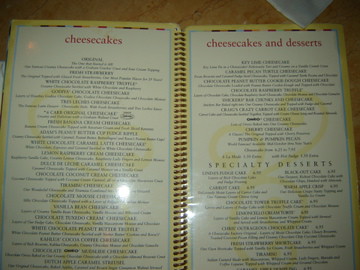In the photo, a wooden table serves as the backdrop. In the upper right corner, part of a napkin is visible, with an opened menu placed just below it. The menu, bound by a spiral binder in the center, has white pages featuring a yellow border around the edges. The pages are vertically aligned and rectangular. On the left page, at the top in red text, the word "Cheesecake" is prominent, followed by a line of text below it, comprising an entire page that is difficult to read even when zoomed in. The right page begins with the heading "Cheesecake and Desserts" in red at the top, followed by half a page of unreadable text. Below this section, the heading "Specialty Desserts" appears, accompanied by another half page of text that is also too small to decipher.